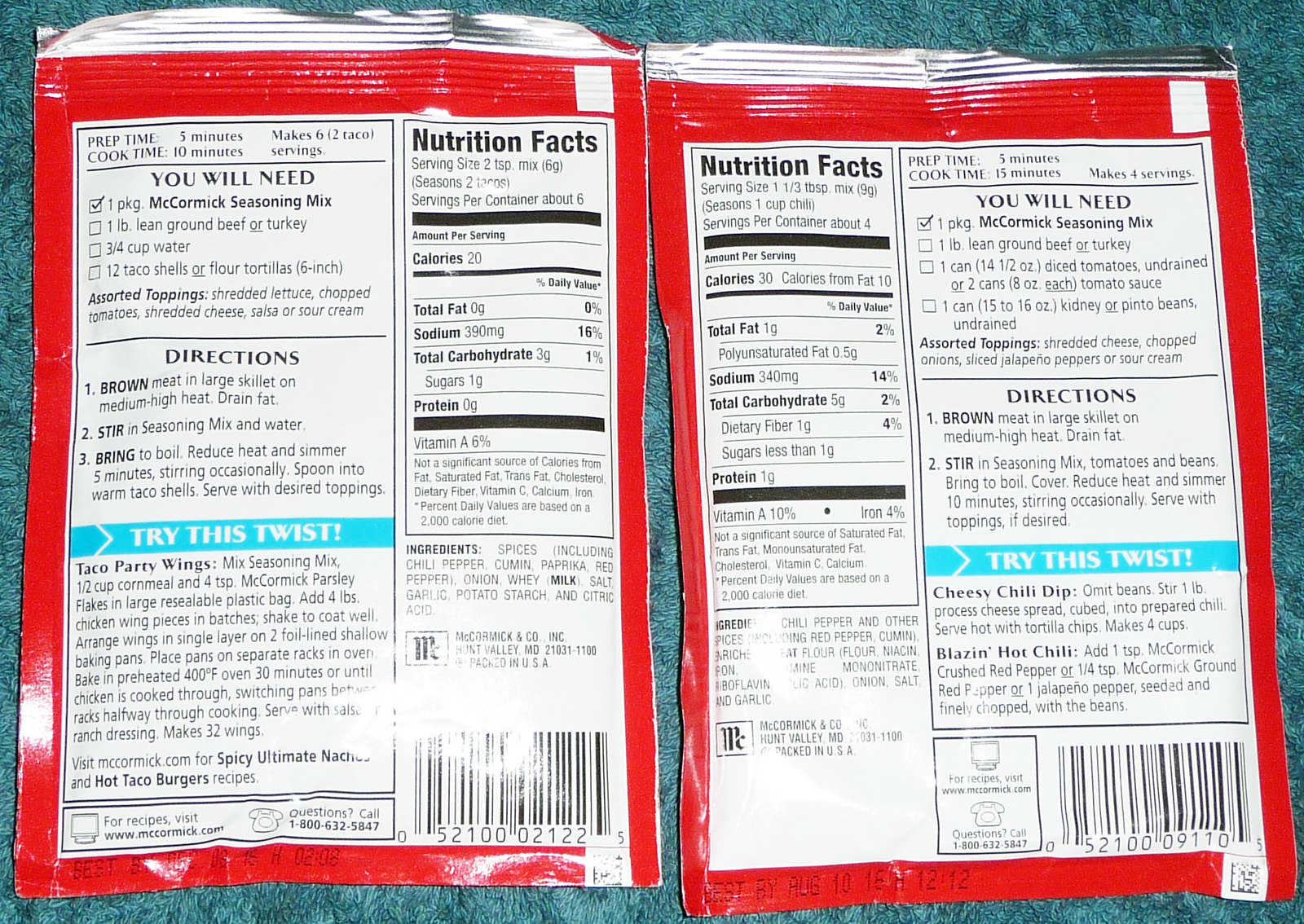Two identical-looking bags of food, possibly chip bags, are laid flat on a greenish-aquamarine rug. Both bags have their backs facing upwards, showcasing their identical packaging. The only noticeable difference between the two is the positioning of the nutrition facts labels; where one label is typically found on the left side, on the other bag, it's on the right. As a result, when the bags are placed next to each other, the nutrition facts labels align side by side. Additionally, the backs of both bags display a set of instructions labeled "You will need to make this bag," presumably offering guidance on how to consume or prepare the contents inside. The greenish hue of the rug contrasts with the vibrant colors of the packaging, making the image visually striking.